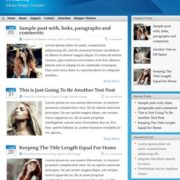Screen Capture of a Web Page Design: A Detailed View

This image portrays a screen capture from an unidentified web page, showcasing a white background that forms the overall canvas of the site. Prominent at the top is a distinct blue horizontal bar serving as a navigation or header section. Directly beneath this bar, there are several menu options displayed in black text, although the text itself is quite blurry and difficult to decipher.

The main content area is divided into two sections. On the left, there is a vertical column featuring three stacked images. The top image displays a blurry photograph of a woman dressed in a brown and white top. Beneath this, the second image features a blonde woman, her head slightly turned to the side with her chin lifted. Finally, the third image shows a woman leaning sideways, although the details remain indistinct due to the blurriness.

To the right of each image, there are accompanying blocks of text, presumably providing context or descriptions for the images. However, the blurriness of the screen capture renders the text unreadable, making it challenging to determine the exact content or purpose of the web page.